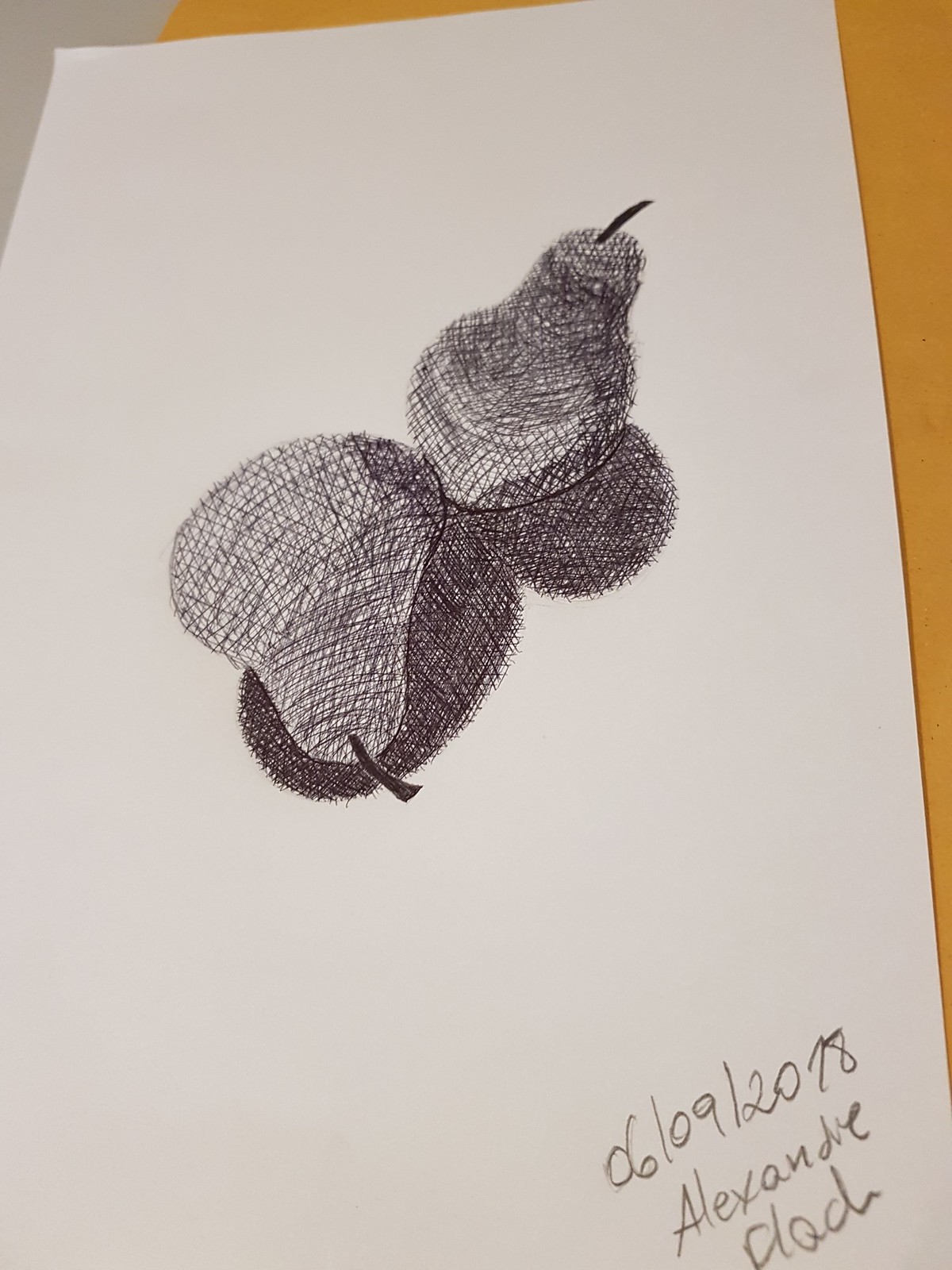On a clean white piece of paper dated 06/09/2018 with the name "Alexander Dad" inscribed at the bottom, the artwork prominently features two pears. One pear stands upright towards the right side of the paper, casting a sharp black shadow underneath it. The other pear lays down towards the bottom of the composition, also accompanied by its own shadow. The shadows, meticulously drawn, provide a striking contrast against the pristine white background, highlighting the meticulous attention to detail in the shadowing and the texture of the pears.